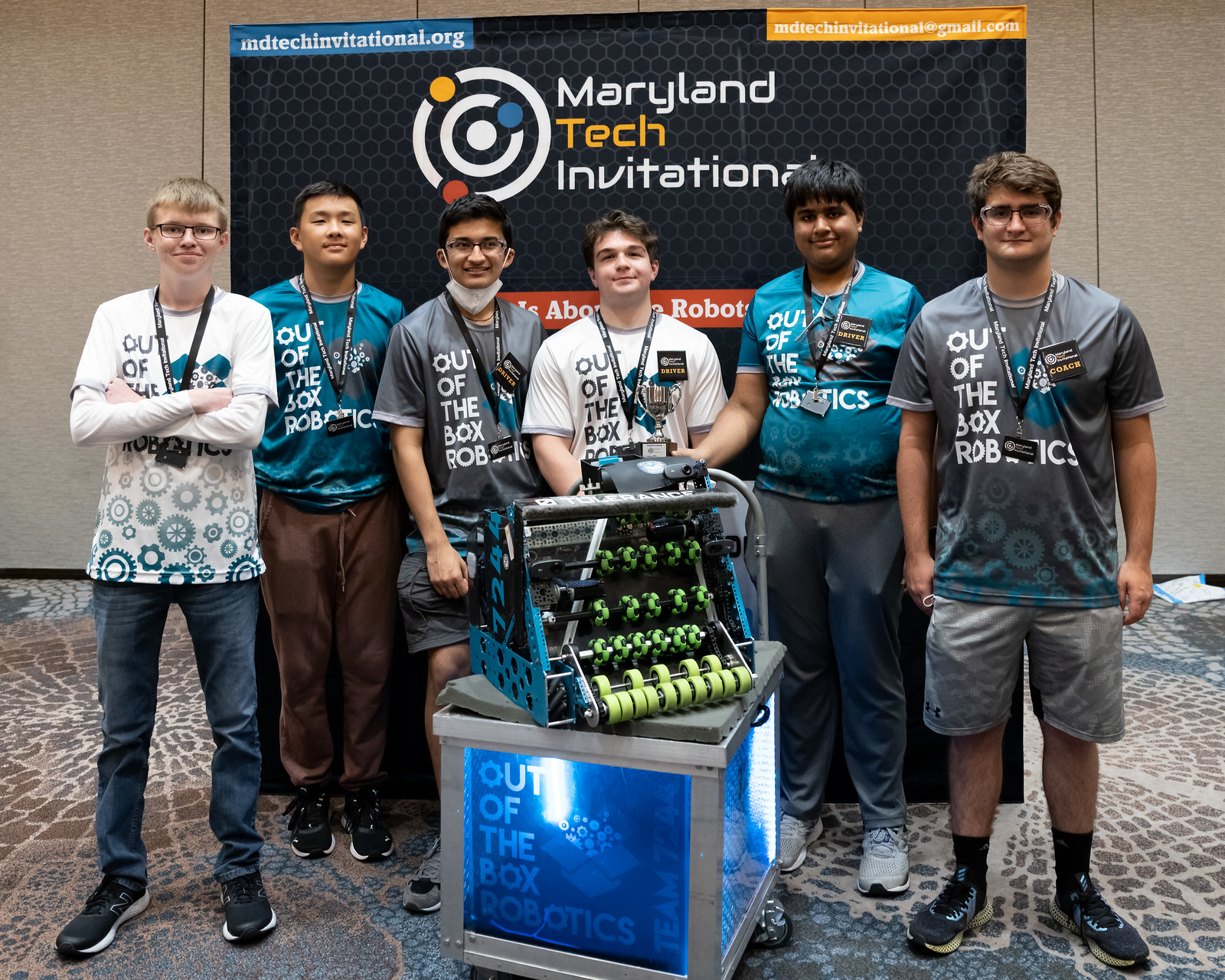This photograph captures a team of six high school students proudly standing behind their invention at the Maryland Tech Invitational. The backdrop features a prominent banner with the event's name, ntechinvitational.org, and contact information. All team members wear lanyards and matching "Out of the Box Robotics" t-shirts in different colors, including gray, white, and teal. From left to right, the students stand in relaxed poses: the first is a white student with short hair and glasses, wearing a white t-shirt and blue jeans; next, an Asian student with short black hair in a blue t-shirt and brown trousers; followed by an Indian student with glasses, a face mask hanging from his neck, gray shorts, and a gray t-shirt; another white student appears partially visible in a white t-shirt; beside him stands another Indian student with a blue t-shirt, gray trousers, and a paunch; and finally, a white student with brown hair and glasses wearing a gray t-shirt, gray shorts, and a badge that reads 'Coach.' In front of them, a complex robot adorned with green wheels, levers, and rods sits atop a large silver box displaying "Out of the Box Robotics Team 7244." One student proudly holds a small trophy above the machine, symbolizing their achievement in the robotics competition.